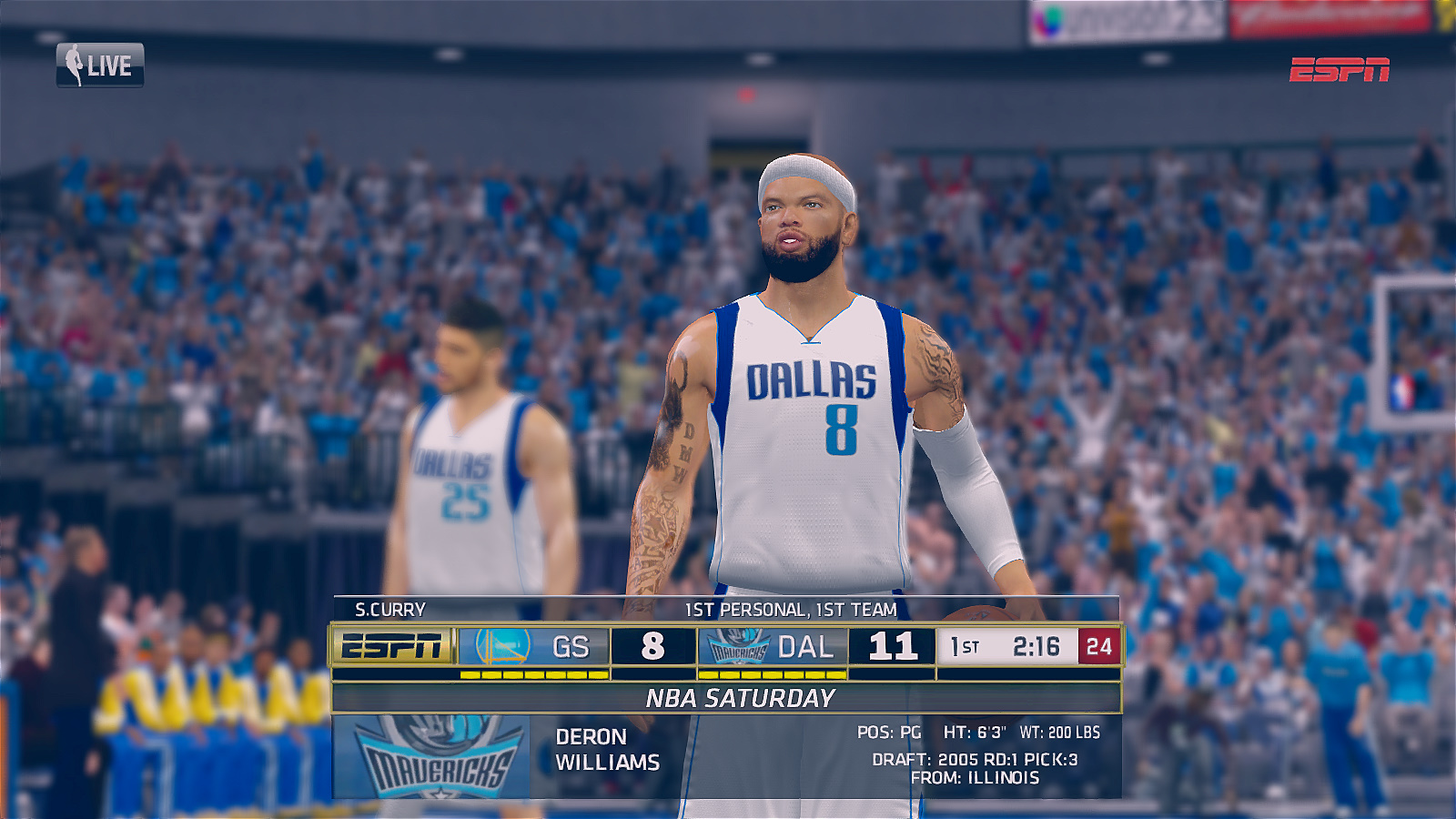This image is a detailed screenshot from what appears to be an NBA video game, possibly NBA 2K, featured on Xbox or PlayStation. The scene depicts a lively gymnasium atmosphere with a realistic-looking crowd, dressed in blue, white, and red shirts. In the foreground stands a player wearing a Dallas Mavericks jersey with the number 8, indicating he is Deron Williams. He is characterized by his tattoos and lifelike appearance, consistent with high-quality video game graphics. 

Adjacent to him is another Dallas Mavericks player, bearing the number 25 on his jersey. The scene highlights an ongoing game between the Golden State Warriors and the Dallas Mavericks, with Dallas leading 11-8 in the first quarter, as indicated by the scoreboard. Above the court, multiple UI elements are visible: the game clock showing 2:16 with a shot clock of 24 seconds, ESPN branding in the top right corner, and a 'live' status in the top left.

Additionally, a detailed player profile for Deron Williams is displayed, listing his position as PG (point guard), height as 6'3", weight as 200 pounds, and draft information indicating he was the third pick of the first round in 2005 from Illinois. This comprehensive overlay shows Stephen Curry's personal fouls, and the data confirms the game's authenticity and close attention to realism.